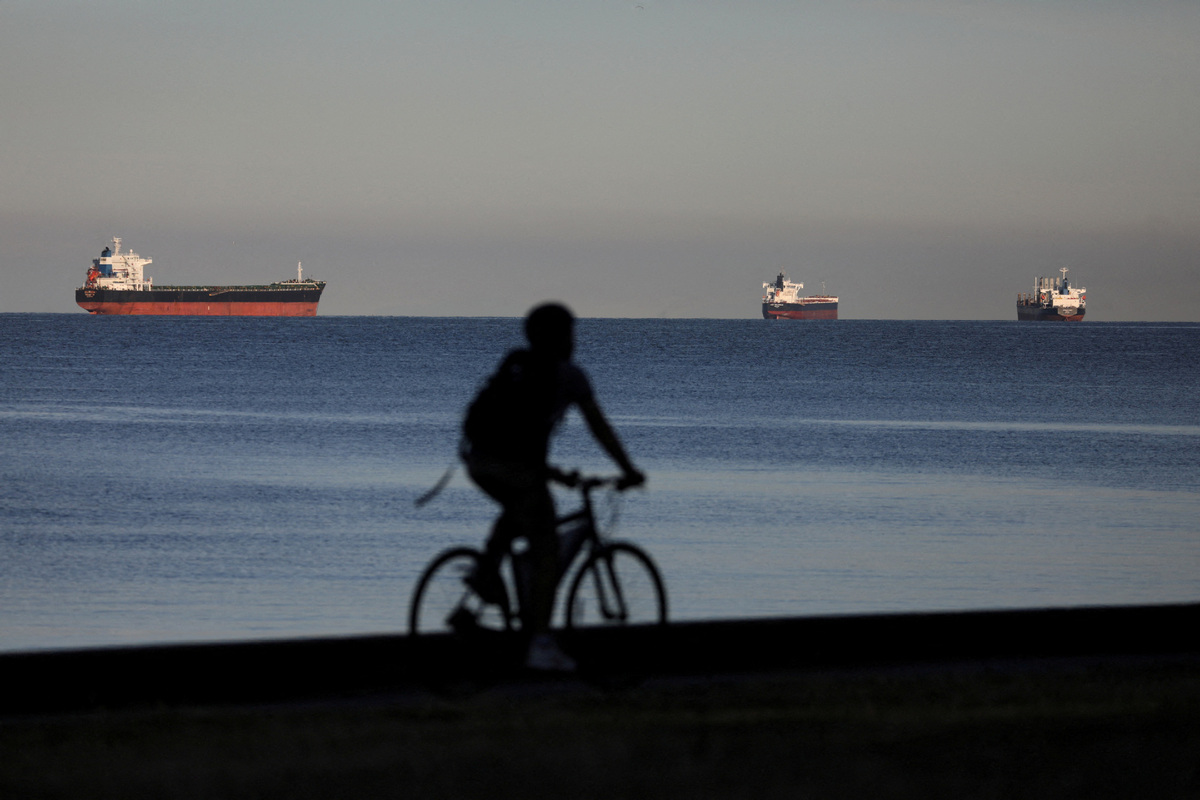The color photograph captures a vivid and serene waterfront scene at either dusk or dawn, bathed in a soft, grayish light. In the foreground, a blurry silhouette of a person riding a bicycle, wearing a backpack and a hoodie, can be seen heading away from the camera towards the right. The clear and calm blue water stretches out behind them, undisturbed by waves. Three very large cargo ships are lined up in the background, two of them appearing empty with a white and brown hue, while the third, colored black and red, seems to be laden with cargo and is sailing towards the left edge of the photograph. The sky overhead is overcast yet cloudless, adding a muted, gray tone to the peaceful scene. There are no other people, animals, or motorized vehicles visible in the image, allowing the focus to remain on the lone bicyclist and the stately ships.